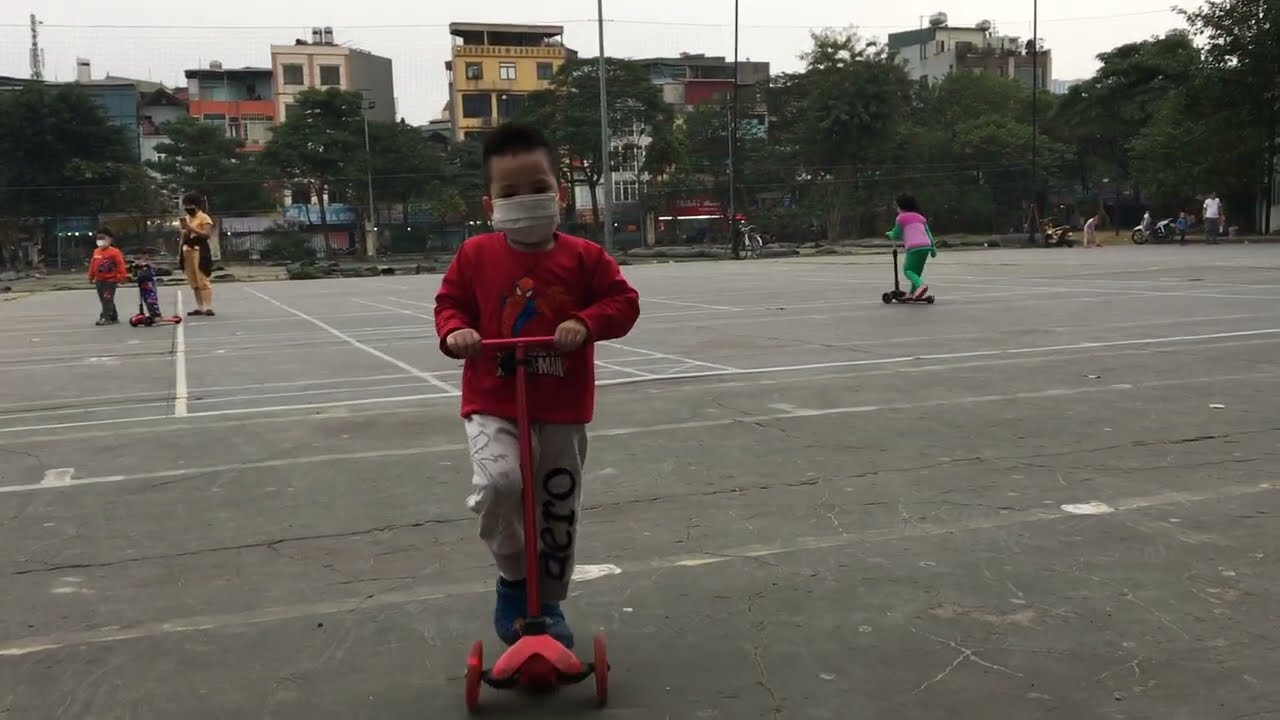The photograph depicts a lively public playground or park, where multiple children are enjoying themselves on red scooters. The central focus is a young boy dressed in a red Spider-Man sweatshirt and pants, looking directly at the camera while riding his scooter. It's an overcast day, and everyone, including the children and a few supervising adults, is wearing COVID-era masks. The rough asphalt surface, marked with white lines, gives the exposed area a somewhat worn-down appearance. Families are present, with some adults capturing moments with cameras. In the background, there are leafy trees and several three to four-story buildings, potentially apartments, hotels, or condos. Also visible are two motorbikes with a couple of people standing next to them. The scene reflects a communal space bustling with cautious activity in uncertain times.